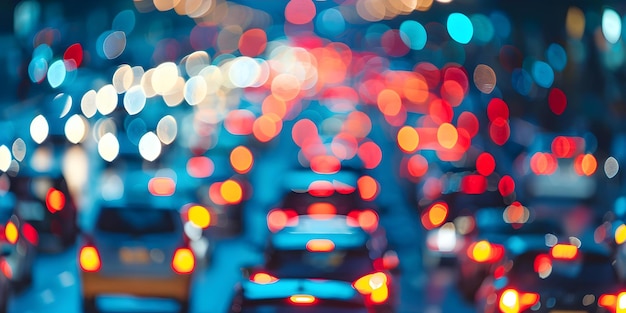The image depicts a scene of heavy, nighttime city traffic, rendered in a surrealistic, heavily blurred manner. The focus is on the vivid, halo-like lights emanating from the cars, predominantly in shades of white, red, and blue, with hints of orange and yellow. These lights form distinct circular patterns that dominate the picture, creating a vivid yet nebulous atmosphere. The white lights populate the left side, transitioning to red in the middle, and culminating in blue on the far right. This specific arrangement lacks an apparent reason but adds to the artistic composition. Although several lanes of cars can be vaguely discerned, individual vehicles are indistinguishable due to the extreme blurriness. The image conjures the sensation of driving at night, particularly with impaired vision, where details are obscured, and lights bleed into one another, forming a radiant, nearly abstract tapestry against a muted, dark blue background. The road and car roofs also mirror this blue hue, further enhancing the overall dreamlike quality of the scene.